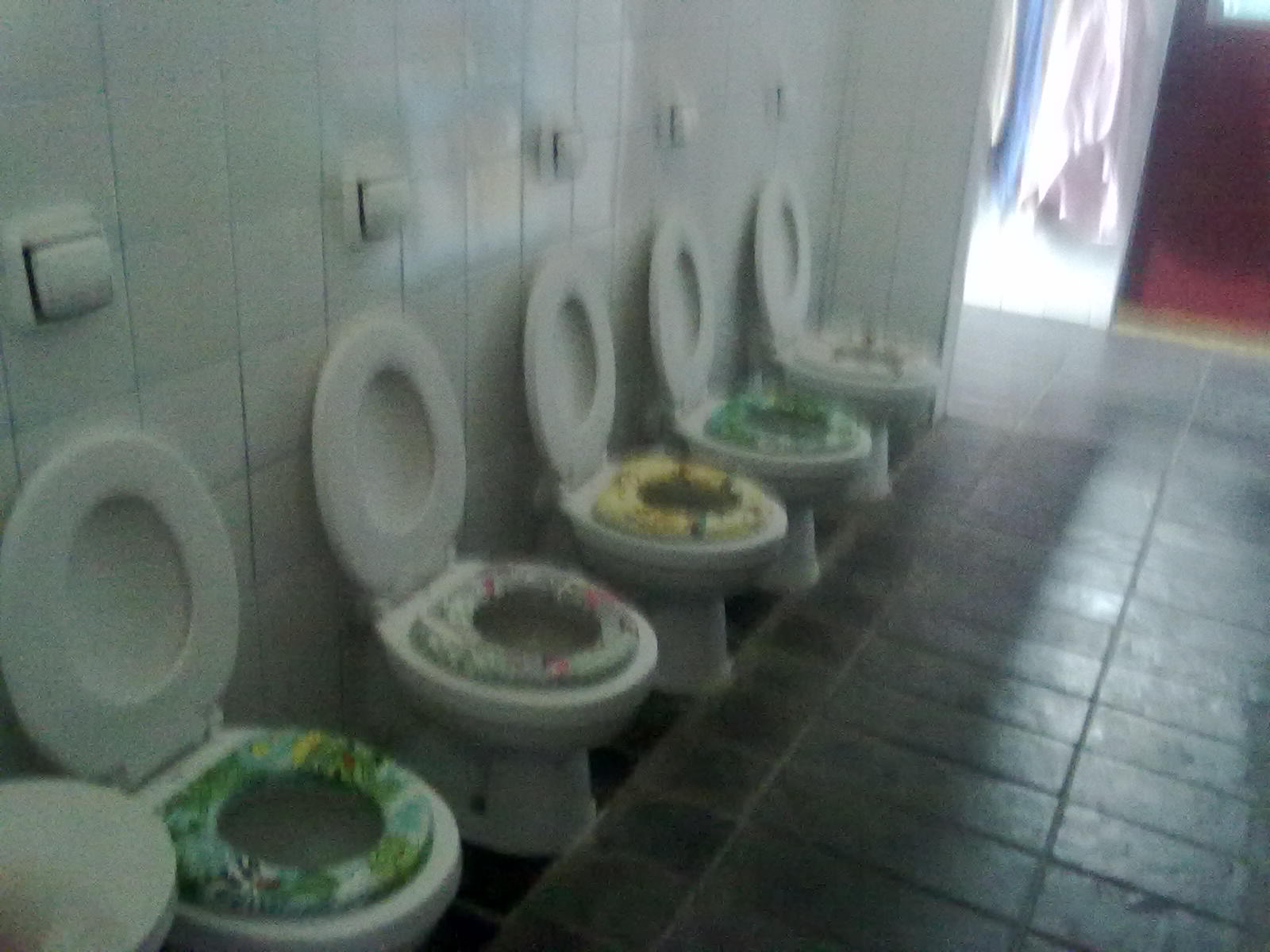The blurry photograph depicts a row of five white toilets lined up against a wall in what appears to be a public restroom. Each toilet has its lid open, revealing uniquely colored and decorated seat designs, including green, white, and yellow variations, which stands out as an unusual feature for such a setting. The wall behind the toilets is covered in white square tiles, adding to the sterile yet somewhat dated ambiance. The dark-tiled floor, combined with the dim lighting inside, creates a stark contrast with a brightly lit area on the right, possibly indicating an entrance or adjacent space. Though the image quality and lighting are poor, a detail of there being a toilet paper roll above each toilet can be vaguely discerned, along with what may be a sink near the first toilet. The overall cleanliness is hard to judge due to the blurriness, but some elements on the toilets could either be intentional decor or signs of unclean conditions.